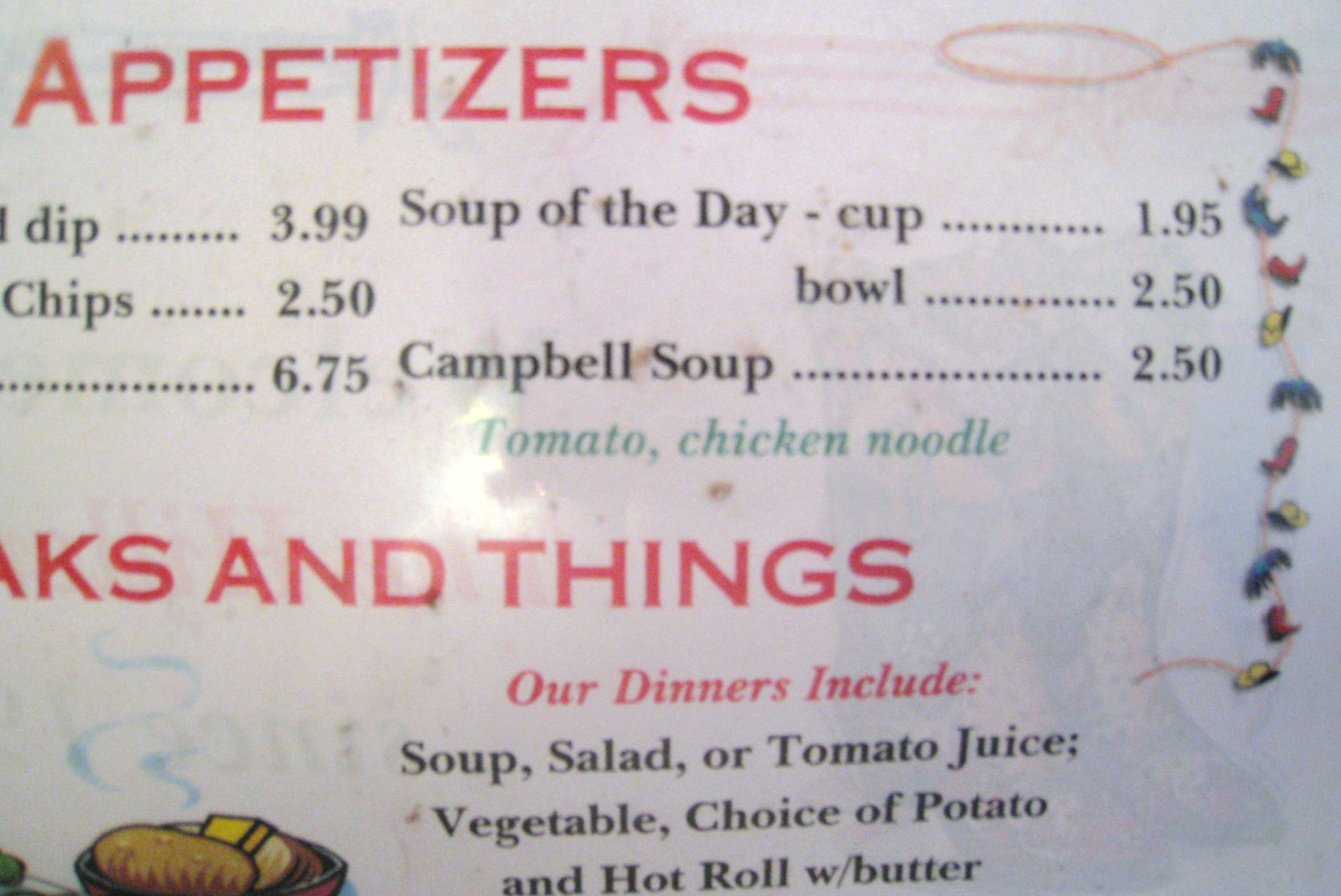The image showcases a glossy white menu prominently featuring the section title "Appetizers" in large red letters at the top. Below, items listed include a dip priced at $3.99, a chips option for $2.50, and another item for $6.75. The menu also offers a variety of soups: the soup of the day is available at $1.95 for a cup and $2.50 for a bowl, while Campbell's soup, priced at $2.50, has choices of tomato or chicken noodle, noted in green letters.

Further down, the menu announces "Drinks and Things" in red letters, followed by a description of meal inclusions in red letters: "Our dinners include." The items listed in black letters are soup, salad or tomato juice, vegetable, choice of potato, and a hot roll with butter.

To the left of this text is part of an image of a plate. The visible portion reveals a large roll, something yellow, and a substantial piece of meat. The plate emits small tendrils of blue-colored steam, giving a sense of warmth and freshness. In the background, tall cowboy boots in shades of yellow and brown add a rustic touch to the scene.